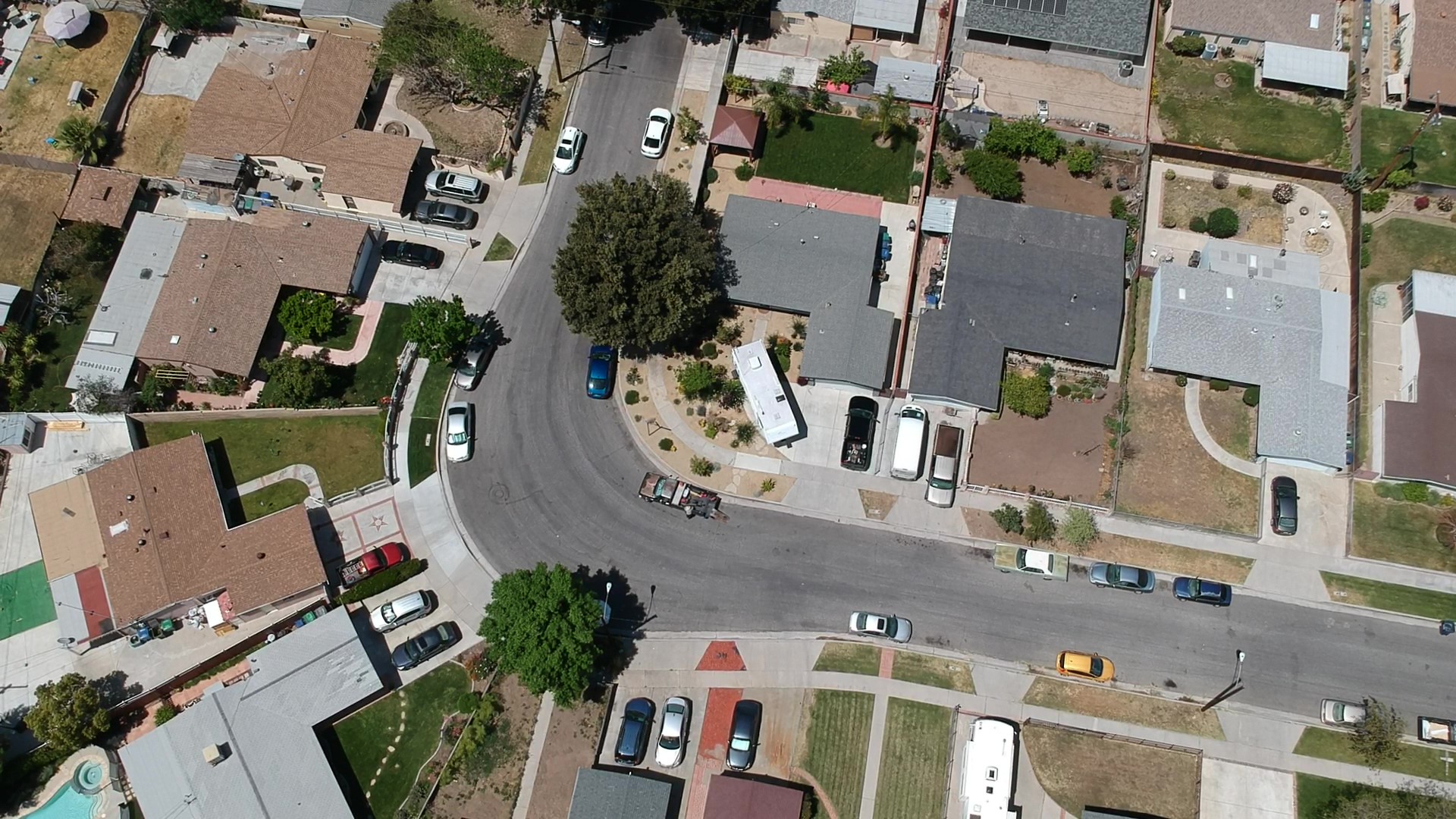This aerial photograph captures a detailed view of a suburban neighborhood, showcasing its residential layout and features. At the heart of the image, a street descends from the top center, gracefully curving to the right before extending straight towards the bottom right corner. Lining the street are several single-story houses, each equipped with garages. Vehicles are parked along both sides of the street and in the driveways.

On the left side of the photograph, four rooftops are clearly visible. The top three houses have brown roofs, while the house in the bottom left corner features a lighter gray roof. This bottom-left property also boasts a swimming pool in its backyard. The yards present a mix of green and dead grass, adding texture and contrast to the scene. Overall, the image provides a comprehensive and detailed glimpse into the suburban setting, highlighting the arrangement and condition of the homes and their surroundings.